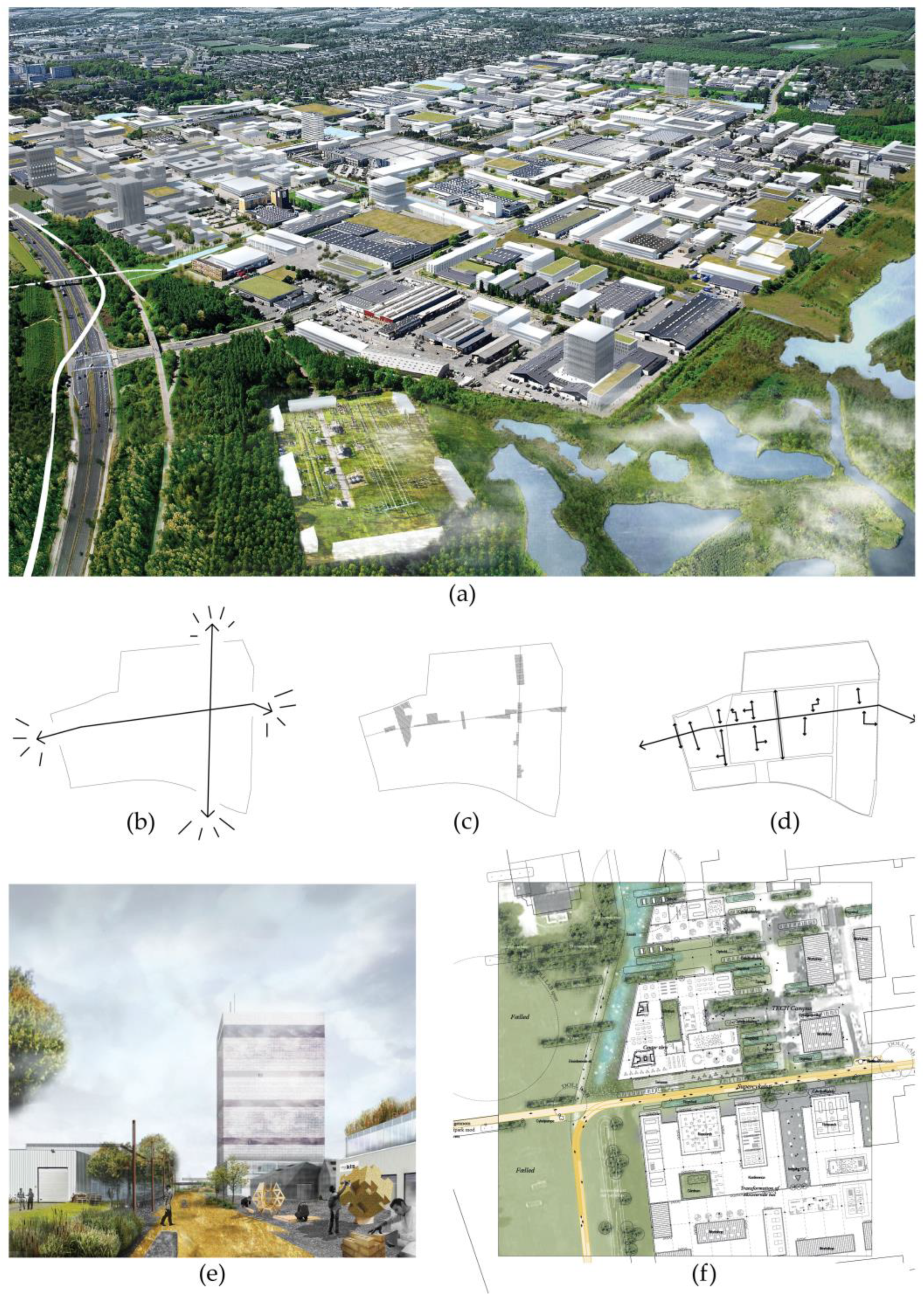The image is an elaborate, multi-layered project proposal for a planned development. At the top of the layout, there is a large aerial photograph showcasing a blend of real and conceptual elements. On the left side, a highway curves around a greenbelt and a series of ponds or pools. Adjacent to this highway is a proposed city development featuring numerous white-roofed commercial buildings with ample parking space. The far background, towards the top of the image, merges seamlessly into an existing urban area with residential and commercial structures surrounded by greenery, indicating a transition from reality to design.

Beneath this primary photo are three diagrams on a white background, labeled B, C, and D. Diagram B shows an outlined plot of land, while Diagram C details the same plot with indicated roadways and gray-marked small land plots. Diagram D further refines this with more defined roadways and a black line with arrows marking specific routes.

In the lower left is Figure E, which presents a street-level view, showcasing a building against a blue sky, possibly depicting the proposed architectural style. The lower right, labeled Figure F, contains a detailed floor plan or blueprint, illustrating the planned city layout within the plot of land. Each element collectively provides a comprehensive view of the proposed development, blending actual geographic features with visionary urban planning.